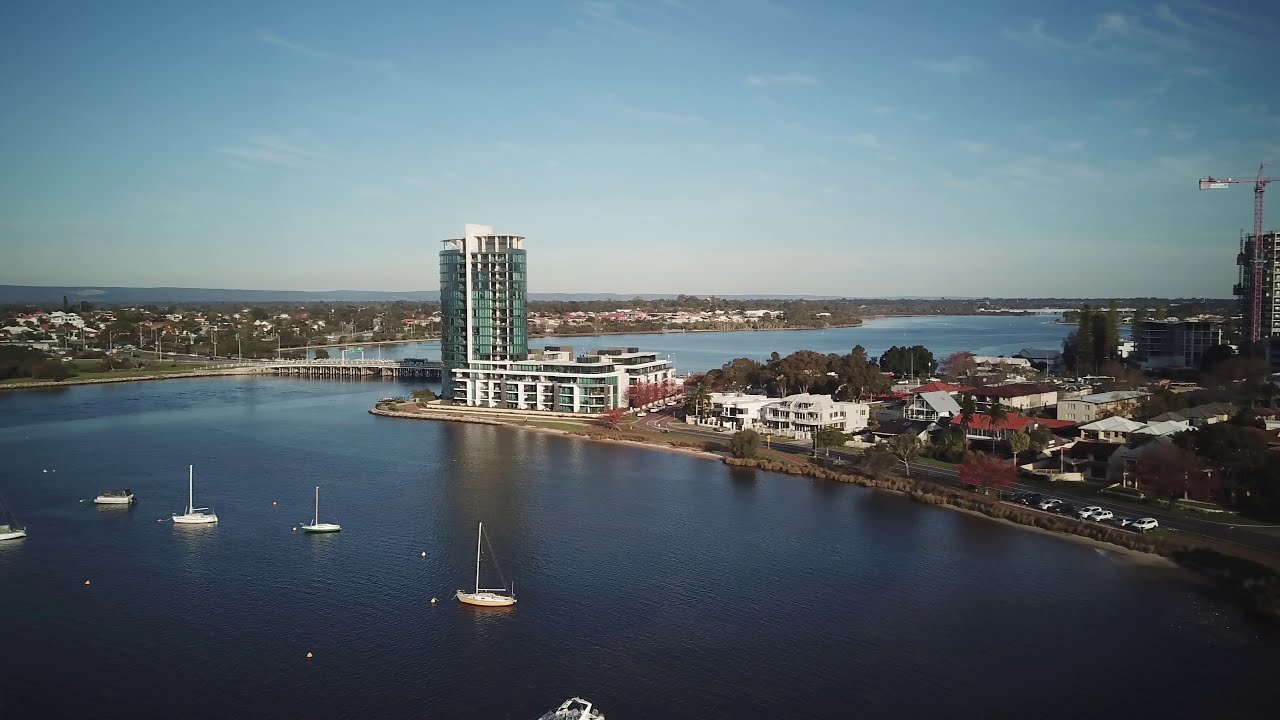The image captures a large, wide river coursing through a cityscape on a sunny day with a light blue sky dotted with small clouds occupying the upper third of the frame. To the lower left, several sailboats without their sails are congregated near a shoreline that features a mix of housing and abundant greenery. Prominently visible on the left shore is a portion of land jutting out into the water, adjacent to a very tall glass skyscraper that resembles a parking garage or an apartment building. A bridge connects this side of the river to the right shore, where there is ongoing construction marked by a crane near the far edge. The right side of the image also shows more homes, parked cars, and trees. Overall, the setting is bright and bathed in natural light, providing a clear, picturesque view of the river and the surrounding urban landscape.